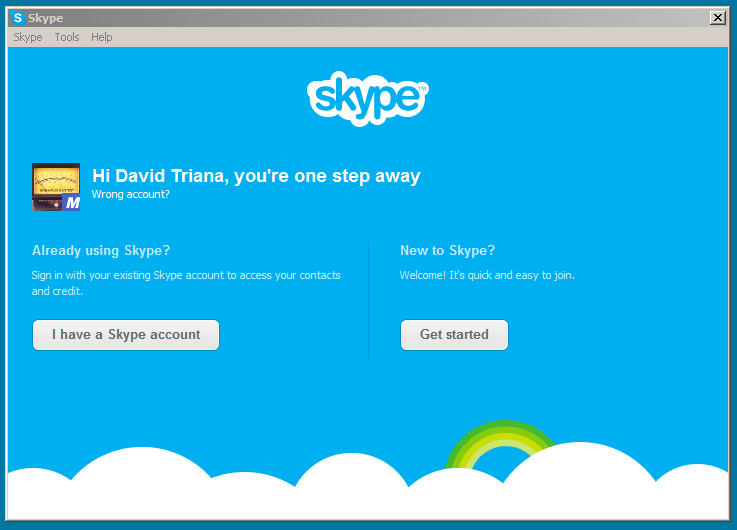The image is a screenshot of the Skype login page. In the upper left-hand corner, there is a gray box containing the Skype logo – a white "S" inside a blue box – accompanied by the word "Skype" in light gray text. Extending from left to right across the screen is a thin gray bar, which is immediately below the logo and contains menu options: Skype, Tools, and Help.

The main window of the screen displays the Skype interface prominently. At the center, the word "Skype" is visible with a blue background. The lower portion of the image features a stylized graphic with the top of a cloud stretching horizontally from left to right, covering the entire bottom. A vibrant rainbow arcs above the cloud, adding a colorful element to the scene.

Text within the main window indicates that this is the login page for Skype. There is an option to sign in with an existing account, alongside another button on the right side labeled "Get started," intended for new users who want to create a Skype account.